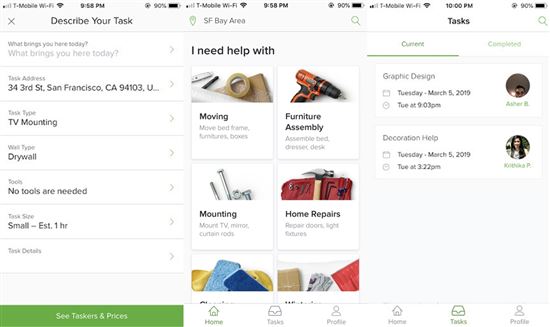This set of images appears to be details from an application used for hiring taskers for various services. Below is the enhanced and detailed descriptive caption:

---

This sequence of three screenshots provides a comprehensive overview of a task booking process through a service application. The first screenshot, captured at 9:58 PM, outlines a specific task titled "Describe Your Task." Key details include:

- **Task Address**: 34 3rd Street, San Francisco, CA 94103
- **Question Prompt**: "What brings you here today?"
- **Task Type**: TV Mounting
- **Wall Type**: Drywall
- **Tools Required**: No tools needed
- **Size**: Small
- **Estimated Duration**: 1 hour (EST.)
At the bottom, a button labeled "See Taskers and Prices" is visible.

The second screenshot, also time-stamped at 9:58 PM, displays options for the user's task location set in the "San Francisco Bay Area." The prompt "I need help with" features a list of categories including Moving, Furniture Assembly, Mounting, and Home Repairs, with additional options cut off from view.

Lastly, the third screenshot, captured at 10:00 PM, shifts to the "Content" view under the heading "Task." The subsection "Completed" appears, with "Content" underlined, indicating the current tab. Tasks listed include "Graphic Design" and "Decoration Help."

---

This detailed caption offers a clear and structured narrative of the screenshots, facilitating understanding for anyone without prior context.